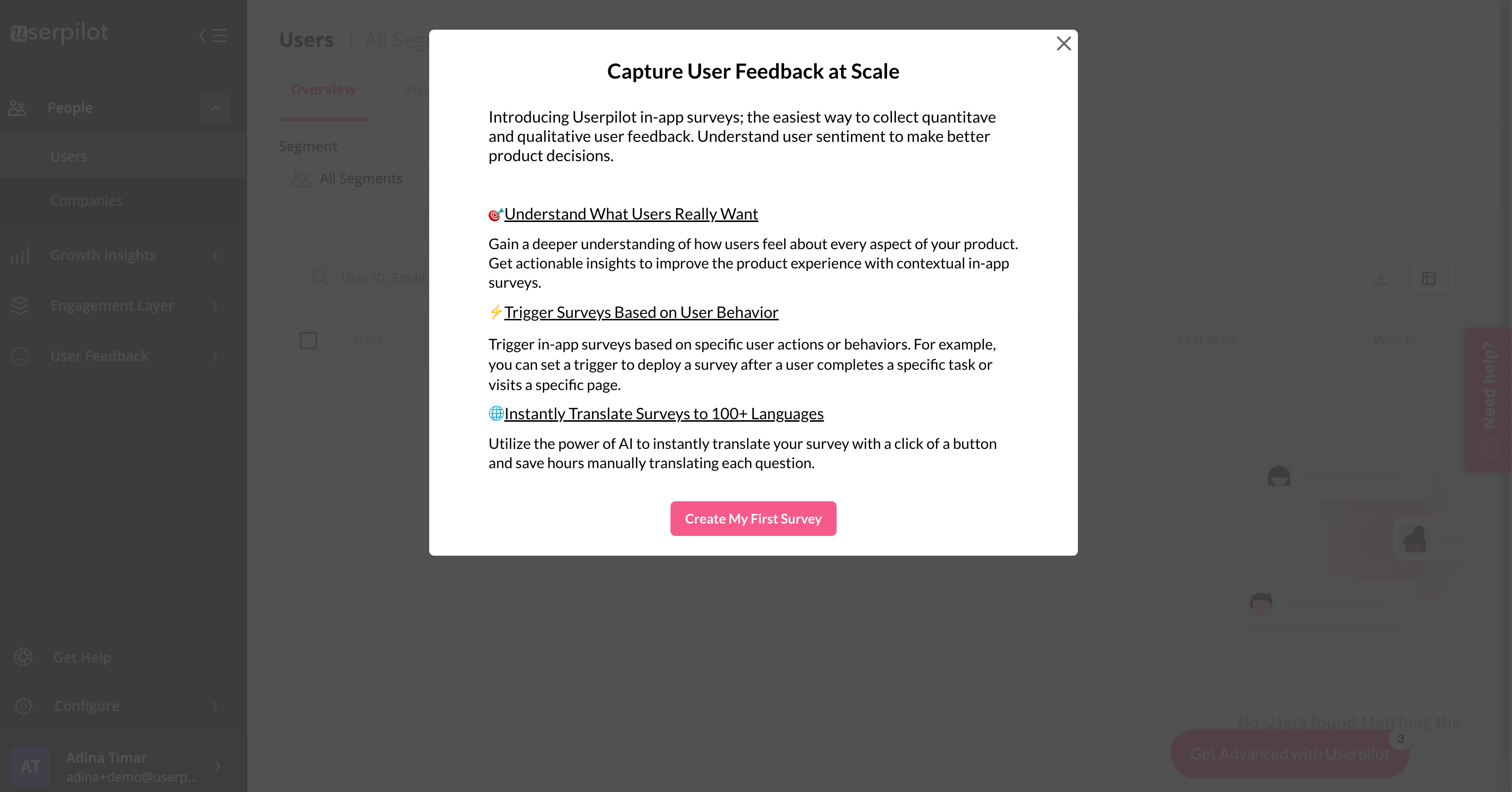The image is a rectangular pop-up window displayed on a dimmed-out screen, commonly indicating that the rest of the background is inactive or less prominent. The pop-up features a white background with a black "X" icon in the upper-right corner, presumably for closing the window.

At the top of the pop-up, bold text reads, "Capture user feedback at scale." Below this headline, a subheading announces, "Introducing UserPilot in-app surveys, the easiest way to collect quantitative and qualitative user feedback. Understand user sentiment to make better product decisions." 

The next section begins with an underlined statement: "Understand what users really want." It elaborates, "Gain a deeper understanding of how users feel about every aspect of your product. Get actionable insights to improve the product experience with contextual in-app surveys."

Another section, also introduced with underlined text, reads, "Trigger surveys based on user behavior." The accompanying paragraph explains, "Trigger in-app surveys based on specific user actions or behaviors. For example, you can set a trigger to deploy a survey after a user completes a specific task or visits a specific page."

The final section, starting with an underlined headline, states, "Instantly translate surveys to 100+ languages." This highlights the feature's multilingual capability, essential for global user engagement.